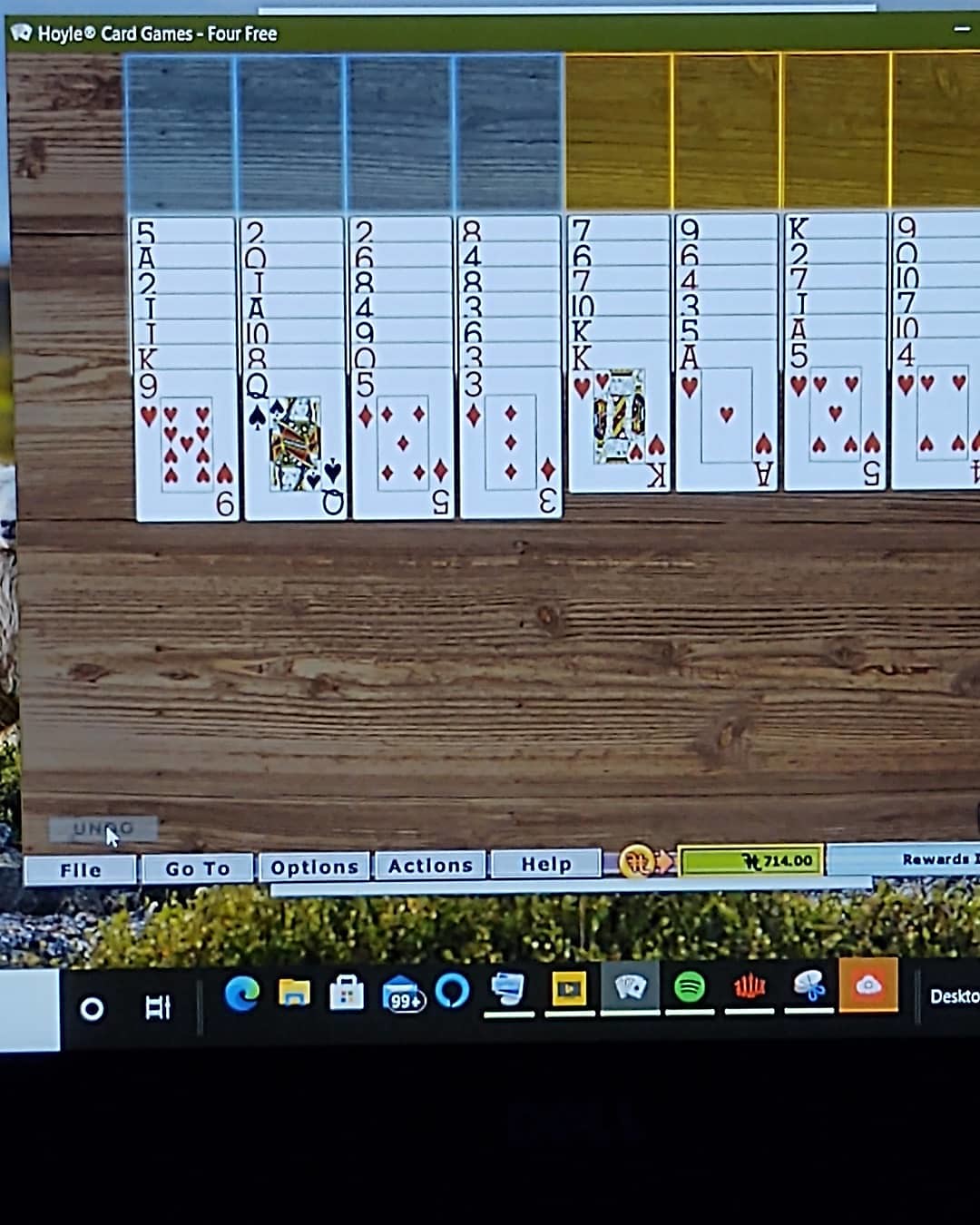In this computerized scene of a Solitaire card game titled "Hoyt Card Games for Free," the game interface is displayed prominently. At the top left corner, the game title is clear and visible. The game board features seven columns of cards. The first four columns on the left each contain seven cards, while the three columns on the right have six cards each, totaling eight layers in height. Beneath the game board, there is a set of navigation buttons labeled File, Go To, Options, Actions, and Help. Adjacent to these buttons, a small yellow display area indicates the score, and next to it, a section labeled Rewards is visible. The bottom of the image hints at it being a computer game, as other icons and applications installed on the user's desktop can be seen.